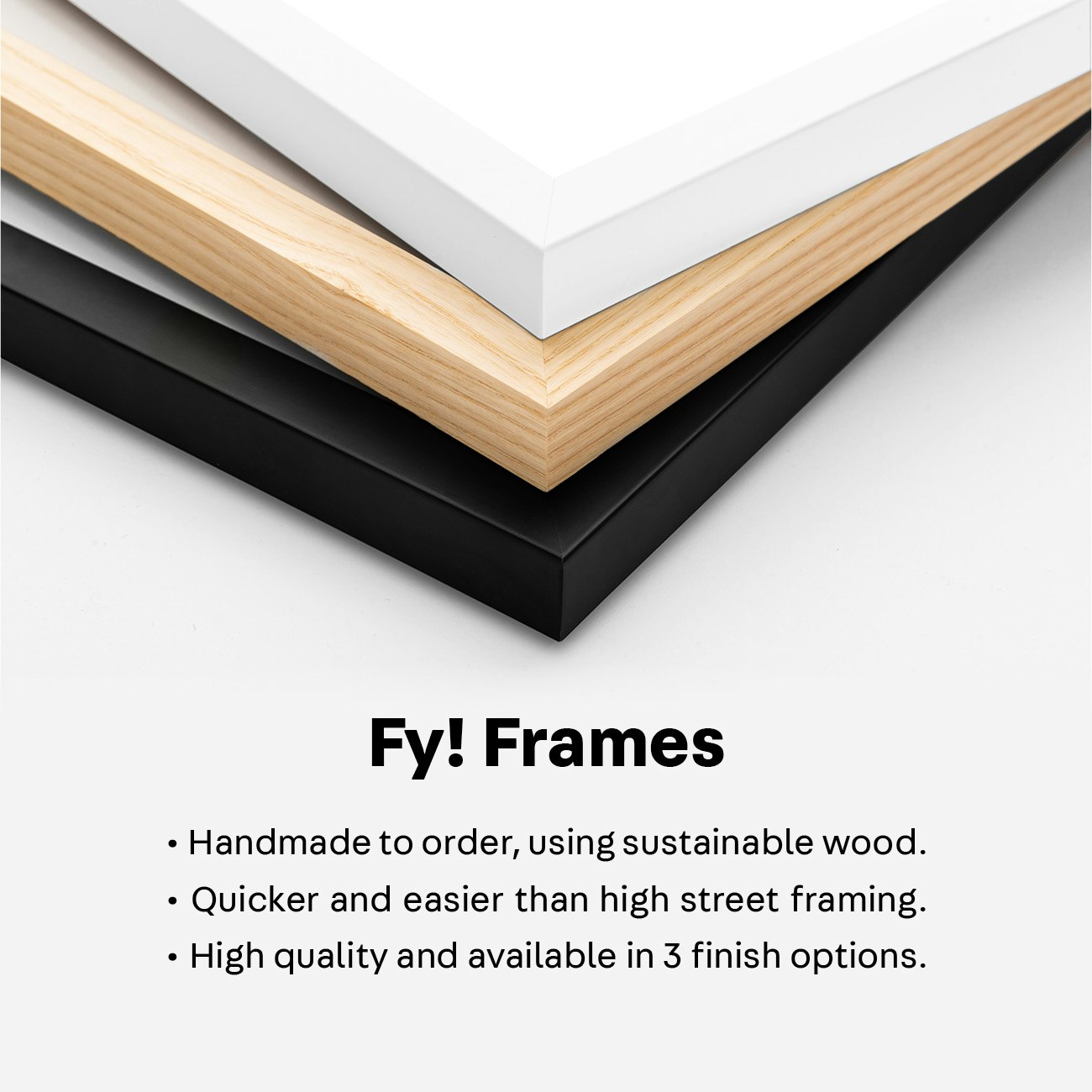The image is a square stock photo showcasing three different picture frames advertised by a company, likely branded as "FY! Frames." The frames are stacked in a cascading manner, each corner pointing towards the bottom center of the image. The top frame appears to be white or possibly light gray, followed by a middle frame of light wood grain, and a bottom frame of black material which could be plastic. The background of the image is a light gray, providing a neutral backdrop that emphasizes the frames. Below the frames, bold black text reads "FY! Frames," followed by three bullet points: "Handmade to order using sustainable wood," "Quicker and easier than high street framing," and "High quality and available in three finish options." Each frame corner is artistically displayed with white matting visible around them, highlighting their distinct materials and finishes.